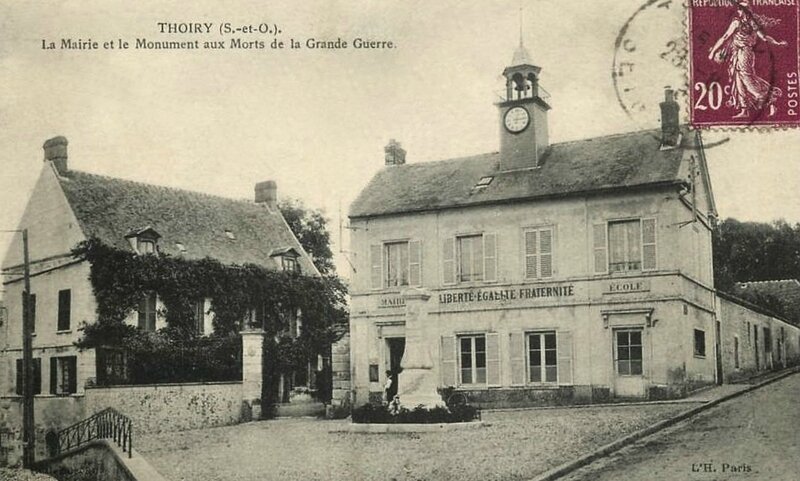This image is an old black and white photograph with a strong feel of a vintage postcard. It depicts a town square in what appears to be a French village. The upper right corner features a maroon postage stamp with a woman’s portrait, marked "20 cents," overlain by a black postmark. In the upper left, the text reads "Thoiry" along with "La Mairie et le Monument aux Morts de la Grande Guerre," indicating that this is a war memorial site. 

The scene captures two primary buildings: the one on the right is a two-story stone structure with an A-shaped roof, a bell tower in the center topped with a circular clock. In front of this building is a courtyard featuring a small stone monument encircled by plants. To the left is another two-story building with a similar A-shaped roof, distinguished by ivy climbing up its facade. The sky stretches above the buildings, and a street can be seen running up the right side of the photo. In the lower right corner of the image, the initials "L-H, Paris" can be seen, suggesting its origin. The overall arrangement of the elements in the photograph is well-balanced, clearly embodying the style of an old, carefully crafted postcard.